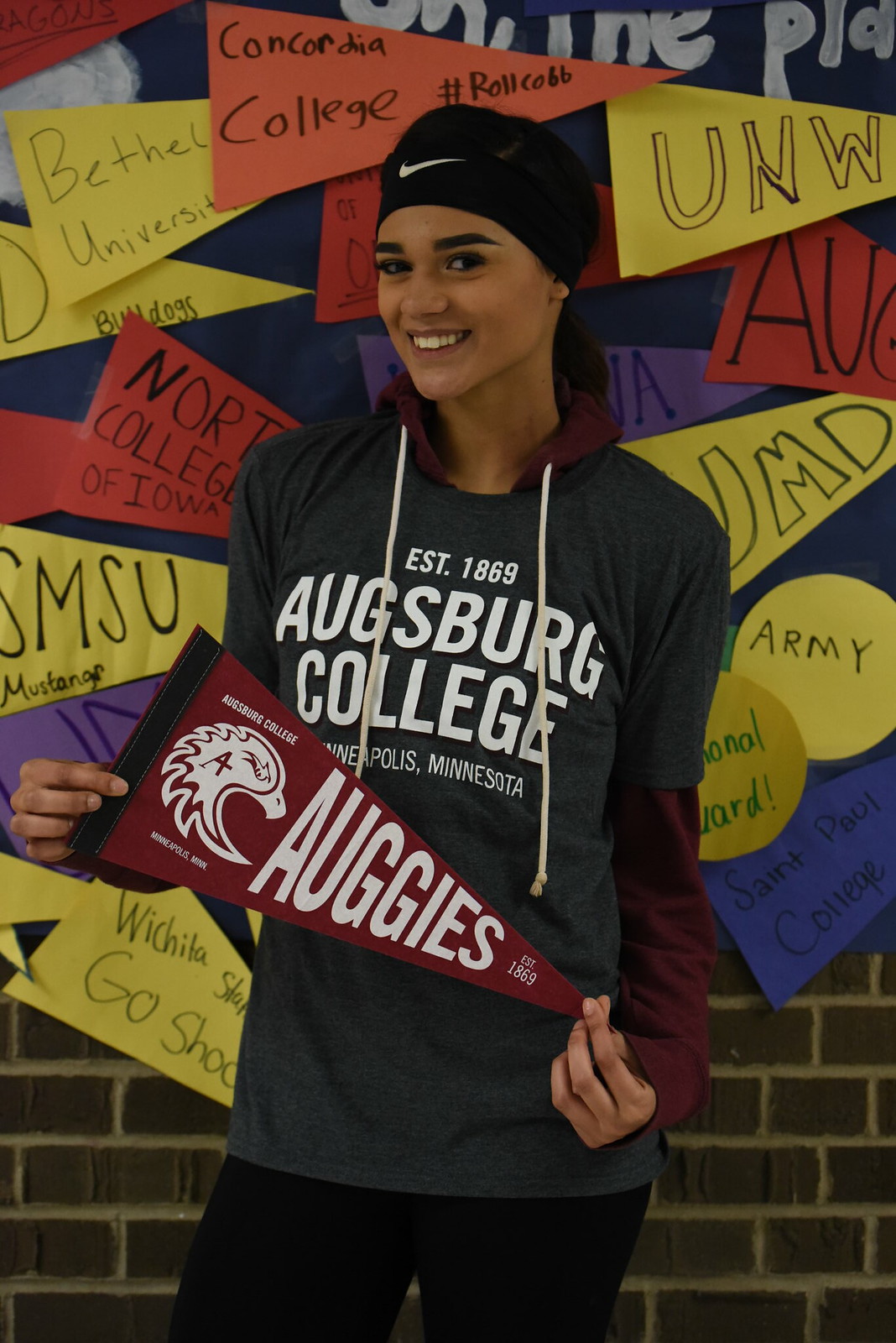The image features a smiling young woman standing in front of a brick wall adorned with numerous hand-drawn and handwritten banners for different colleges, including Concordia College, UNW, SMSU, and the Army. Prominently displayed on the wall are also colorful construction paper flags, hand-crafted without handles. The woman is wearing a long-sleeve burgundy cotton hoodie beneath a short-sleeve dark gray shirt with white writing that reads "Augsburg College, Est. 1869." Over the hoodie, white strings and the hood itself are visible. She accessorizes her look with a black Nike headband. In her hands, she holds a cotton Augie's banner sans handle, featuring a white eagle head icon with an "A" on it, emphasizing her connection to Augsburg College.